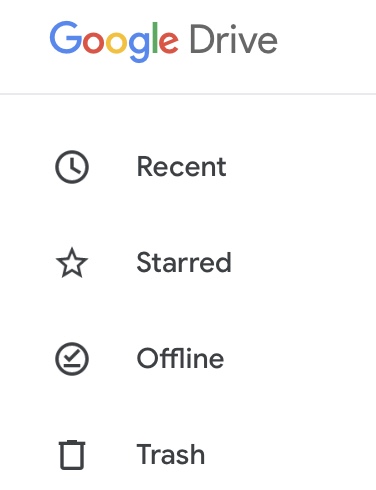A screenshot of the Google Drive website interface displays the iconic Google logo at the top. The Google letters are vibrantly colored, with the first 'G' in green, first 'O' in red, second 'O' in yellow, second 'G' in blue, 'L' in green, and 'E' in red. To the right of the Google branding, "Drive" is displayed in a minimalist gray font against a clean, white background. Beneath the header, a thin gray line provides a subtle separation from the main content below. The primary navigation options are listed on the left side, each marked by a distinct icon: the 'Recent' option accompanied by a clock icon, 'Starred' signified with a star icon, 'Offline' paired with a circle containing a checkmark and line, and finally, 'Trash' indicated by a small trash bin icon.